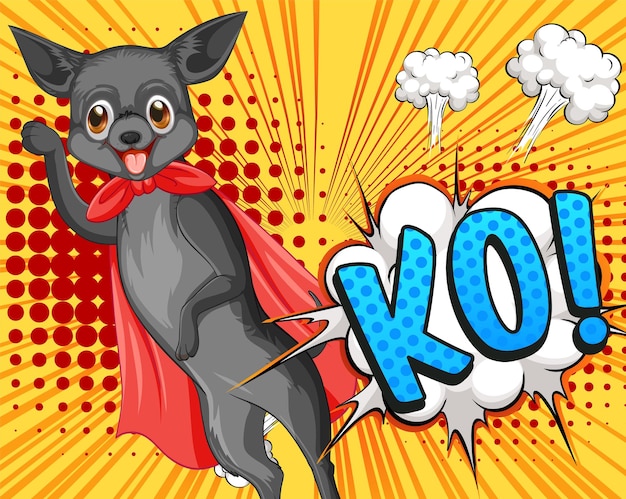This image is a vintage-style comic book illustration featuring a grey dog superhero against a vibrant background. On the left side, the cartoon dog, drawn with large oval brown eyes and a cheerful open-mouthed smile showing its tongue, stands upright on its hind legs. The red cape tied in a bow under its neck flutters out behind it. The dog is posed dynamically, with its left forepaw bent and extending in front of its chest and its right foreleg extending outward and upward as if preparing to take flight.

The right side of the image prominently features a classic comic-style white speech bubble outlined in black, containing the bold text "K-O!" The letters are a light blue with darker blue polka dots and are heavily shadowed to create a three-dimensional effect. Above the speech bubble, there are two additional puffy white cloudbursts, enhancing the dramatic flair of the illustration. The background is a rich mustard yellow with an orange halftone pattern and radiating orange stripes, adding to the retro aesthetic of the scene.